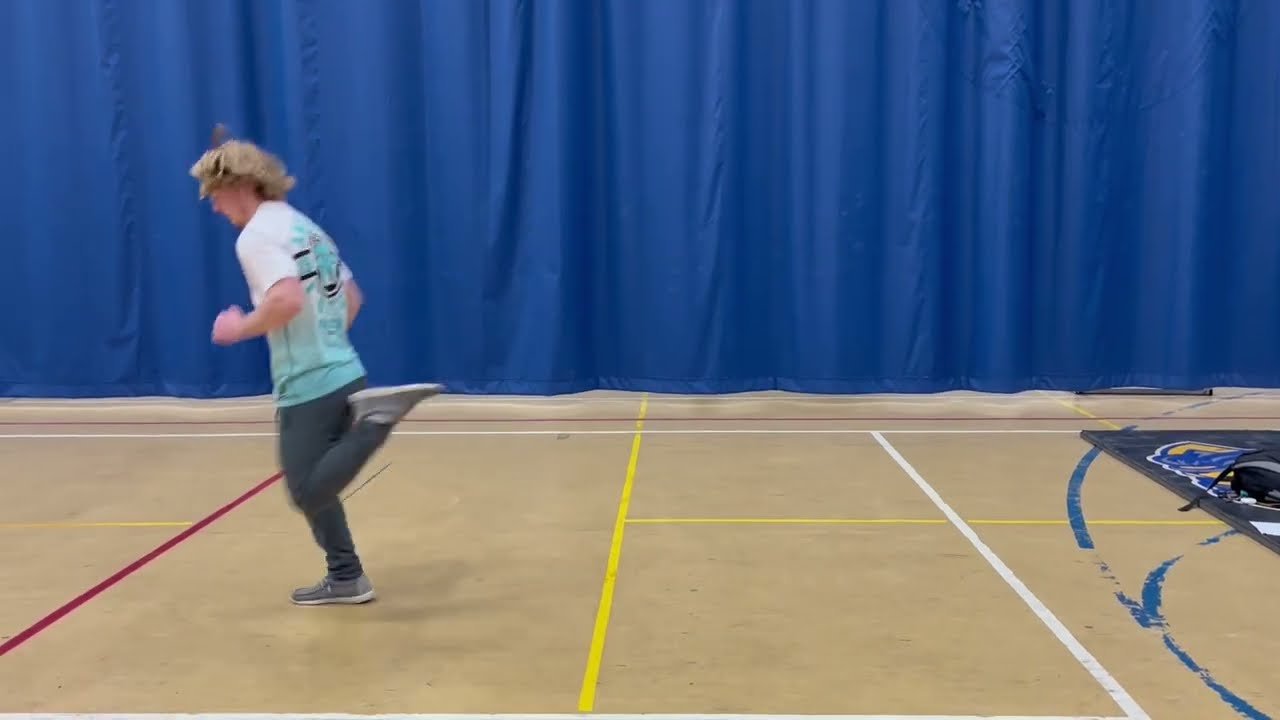The image depicts the interior of a gymnasium, defined by a cream-colored athletic floor marked with various colored lines, including red, yellow, white, and blue, which likely delineate different types of courts, such as for tennis, pickleball, or volleyball. To the right of the floor is a square mark. A blue curtain hangs in the background, suspended from the ceiling, with some portion of the floor extending behind it. In the left-center of the image, a young Caucasian man with long, blonde hair is captured mid-stride while running. He is dressed in gray pants, gray tennis shoes, and a short-sleeved shirt bearing a logo on the back. His arms are raised, and his hair is flying back, emphasizing the rapid motion of his run.